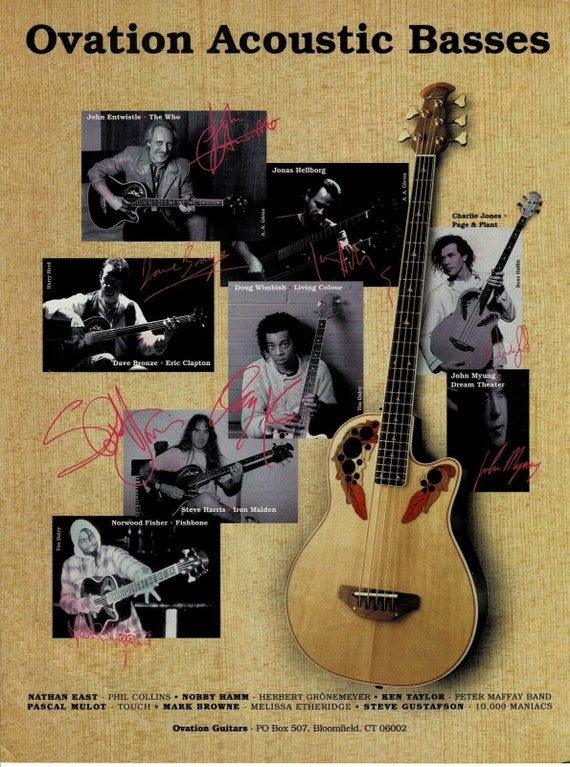The image is a vertically-aligned rectangular poster with a tan, light brown wood-like background. At the top, in bold black letters, it prominently displays the title "Ovation Acoustic Basses." The central part of the poster features a collage of eight black-and-white photographs, each of different prominent musicians playing guitars. Among these, the photo at the center is square, while two vertically-aligned rectangular photos are positioned on the right side.

The musicians featured from left to right and top to bottom include:
- John Entwistle from The Who.
- Jonas Netborg.
- Dave Bronze.
- Eric Clapton.
- Doug Wimbish of Living Colour.
- Steve Harris of Iron Maiden.
- Norwood Fisher from Fishbone.
- Charlie Jones from Page and Plant.
- John Myung from Dream Theater.

Each of these photos has associated white print identifying the musician and their band. Notably, many of the musicians have signed their names on their respective photos.

Positioned to the right of the photo collage is an image of a vertically-standing Ovation acoustic bass guitar. The guitar features a light brown wooden body, gold knobs at the top, and an intricately handcrafted feather-like design on the body.

At the bottom of the poster, in black print, several more musician names are listed, including Nathan East, Nobby Hamm, Herbert Grönemeyer, Ken Taylor, Peter Maffay Band, Pascal Mullet, Mark Brown, Melissa Etheridge, and Steve Gustafson from 10,000 Maniacs. Below these names, it reads "Ovation Guitars" alongside an address, providing further information and context for this promotional poster.